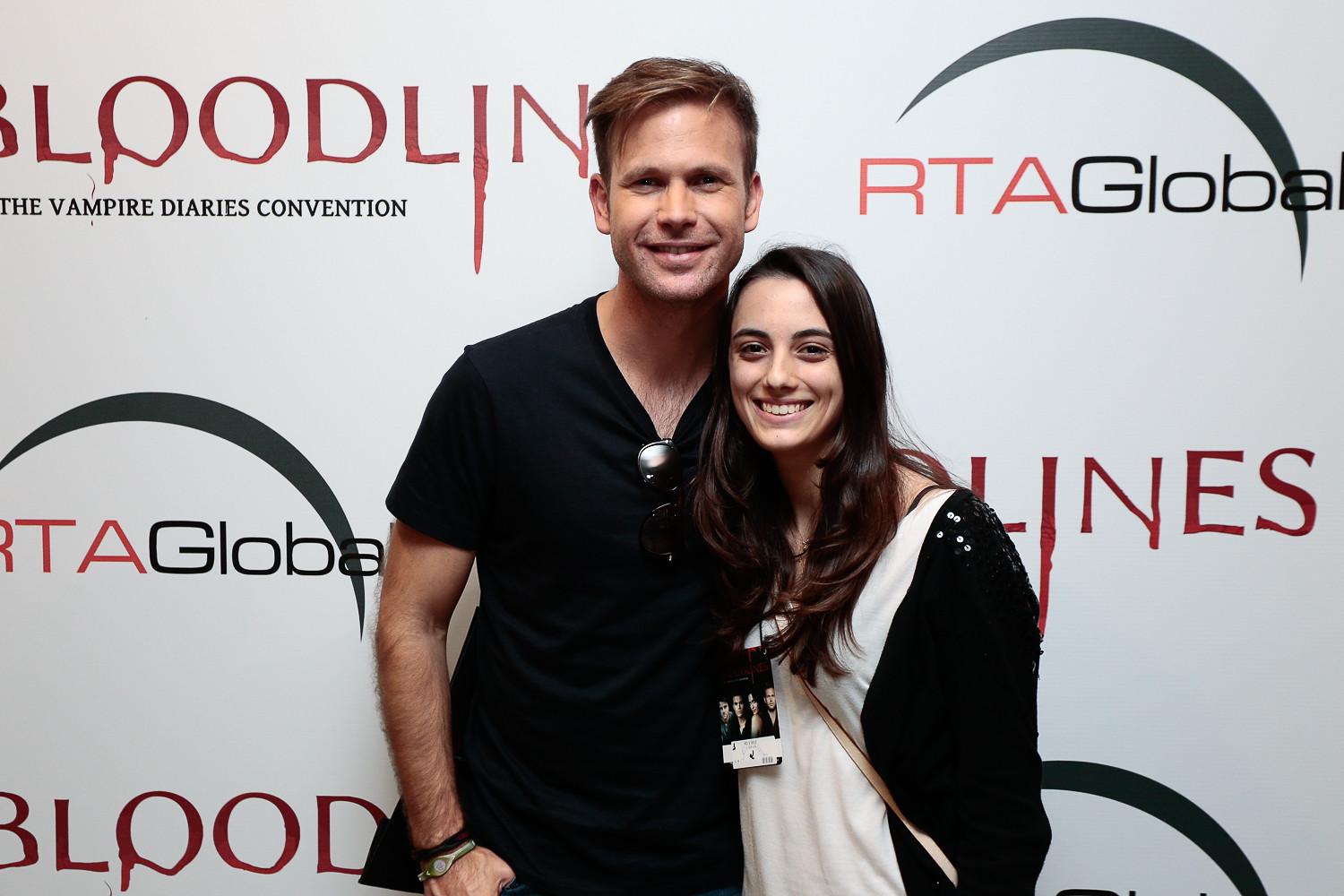In this image, a young man and a young woman stand together, both smiling against a backdrop that prominently features the phrases "Bloodlines," "The Vampire Diaries Convention," and "RTA Global." These elements repeat across the backdrop, with "Bloodlines" in red and "The Vampire Diaries Convention" in black. The word "Bloodlines" is designed with blood dripping from the letters "O" and "I," reminiscent of vampire fangs, and RTA Global appears to be the event sponsor, further hinted by the presence of a crescent moon symbol among the lettering.

The man, who has blondish hair combed to his right, is wearing a black t-shirt with sunglasses tucked into the v-neck and a watch and bracelet. The woman, who has long dark hair flowing over her chest and back, wears a white shirt, a black sequin-adorned jacket, and a lanyard or ID tag hanging around her neck. Additionally, she has a strap across her body, possibly a purse or a backpack. The backdrop and their attire suggest that they might be attendees or participants in the Vampire Diaries Convention.